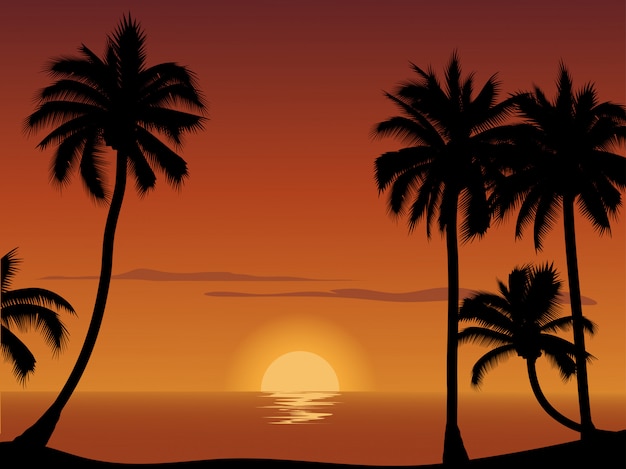This minimalist vector art graphic captures a serene and idyllic tropical sunset over the ocean. The horizon line sits towards the bottom, about 80% down from the top of the image, setting the stage for a dramatic sky transition. The sky is a gradient, shifting from a deep brown at the top through rich oranges to a radiant gold near the horizon. Nestled in the center of the horizon line is a half-set sun rendered in light yellow, with a radial gradient emitting outwards, adding depth and warmth to the scene. The water below mirrors this golden hue, textured with wavy yellow lines that fan out from the point where the sun kisses the horizon, tapering towards the shoreline at the foreground. Silhouetted against this vivid backdrop are five palm trees, their black outlines starkly defining the simple elegance of the scene. Two palm trees stand to the left, and three to the right, with one noticeably curved and about half the size of the others. A faint suggestion of gray streaks punctuates the sky, representing wispy clouds. The combination of these elements—the glowing sky, the dark silhouettes, and the tranquil water—creates a captivating visual experience, perfect for sunset admirers.